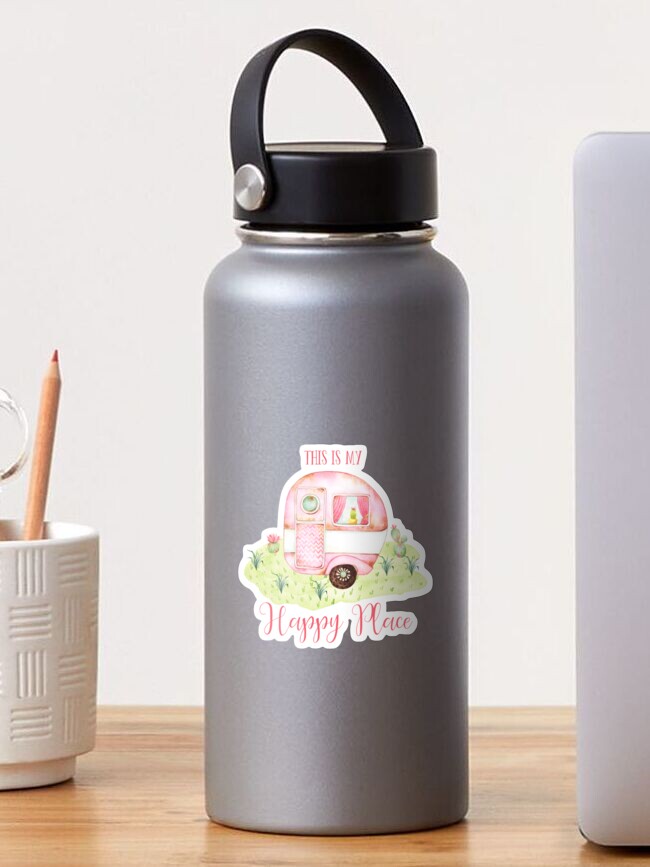The photograph features a dark gray tumbler designed for either hot or cold beverages, centrally positioned on a light wooden table against a white wall. The tumbler has a black rubber lid equipped with a carrying handle secured by a silver grommet. Adorning the front of the tumbler is a vibrant decal with a pink and white trailer, complete with pink curtains in the window and a tiny yellow object on the windowsill. This trailer, which rests on a patch of green grass dotted with darker green flowers and small cacti with pink blooms, has a stubby, single-wheel design. Accompanying the illustration is the text "This is my happy place" in pink, with "This is my" above the trailer and "happy place" below it. To the left of the tumbler, there's a white ceramic mug holding an orange colored pencil, possibly with scissors or another item slightly visible inside. On the right, a smooth, off-white rectangular object, perhaps the edge of a laptop, is partially in view.